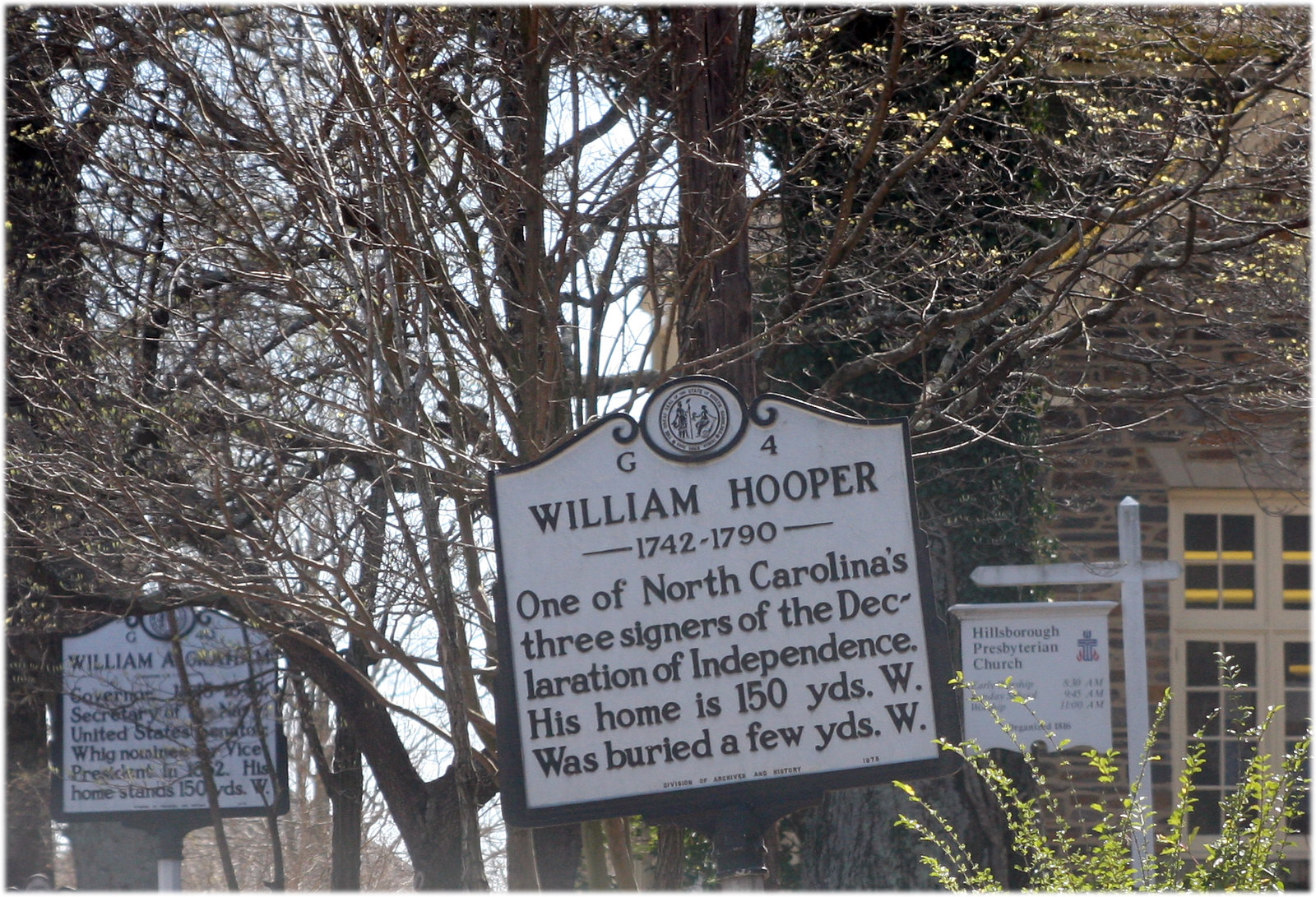This outdoor image captures a large historical plaque affixed to a tree, featuring a black border with a distinct curved top that dips down in the middle, making room for a round circle with an emblem. The text on the plaque is detailed, with "G" on the left and "4" on the right, followed by "WILLIAM HOOPER" in large capital letters. Below his name, the plaque lists the years "1742 / 1790" and continues with the inscription: "One of North Carolina's three signers of the Declaration of Independence. His home is 150 yards west. Was buried a few yards west." This is all on a white background with black lettering.

To the left of this tree, other trees are visible, including another similar plaque in the distance. A building is located not too far behind the tree on the right-hand side of the image, with a window on the right edge and a white pole with a white, unreadable sign slightly behind the main plaque. A hint of greenery tinged with yellow appears in the bottom right corner of the image. The setting is in North Carolina, and the site references indicate proximity to the Hillsborough Presbyterian Church.